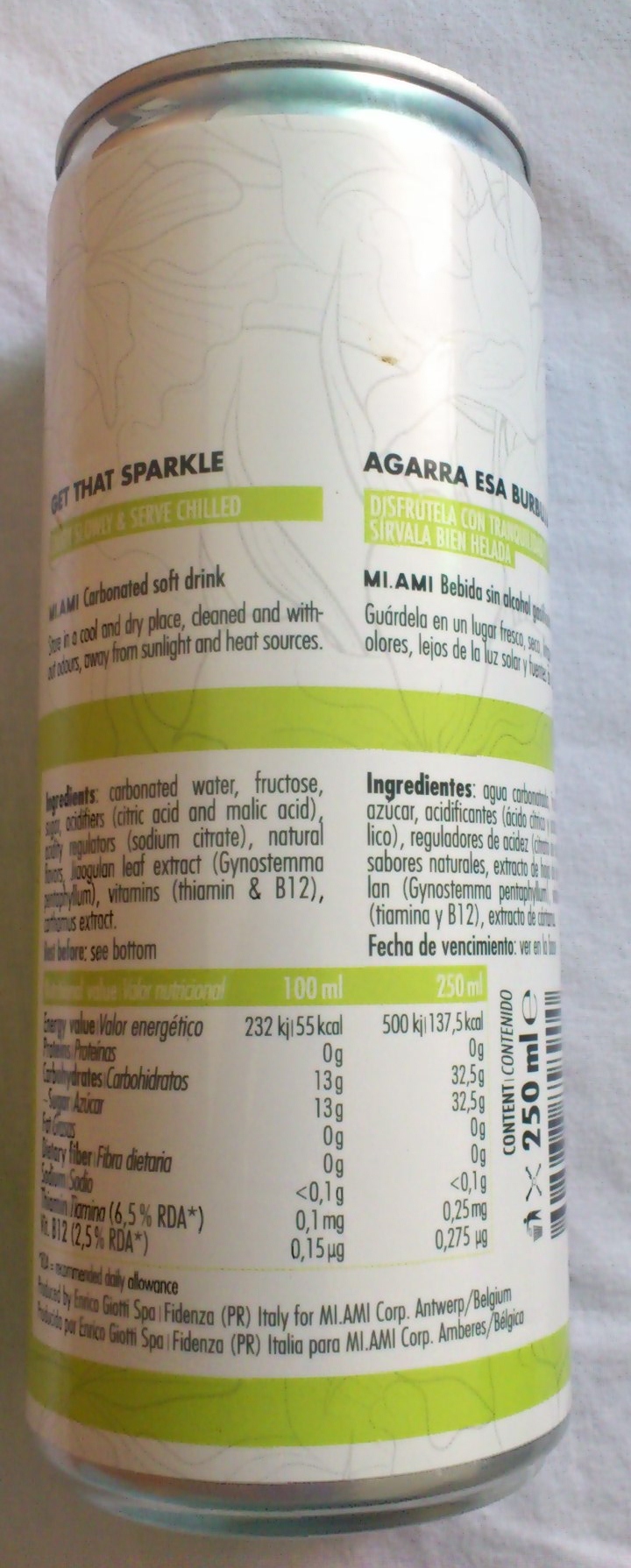Detailed Caption: 

The image features the backside of a slender, white can positioned slightly turned away from the viewer. The can's back displays a wealth of information in both English and Spanish, divided into two columns. On the left side, written in black text, the phrase "Get that sparkle" is clearly visible. Beneath this, a green box contains additional text that appears to promote serving the beverage chilled, although the exact text is partially obscured due to the angle of the can. Further down, the English description includes storage instructions, advising to "Store in a cool and dry place, away from sunlight and heat sources." A list of ingredients follows this storage directive. Parallel to the English text, the right column contains the same information translated into Spanish. The bottom right segment of the can features a logo and a scannable QR code. The can is resting on a smooth, white sheet, which acts as a plain backdrop, drawing focus to the details on the can.